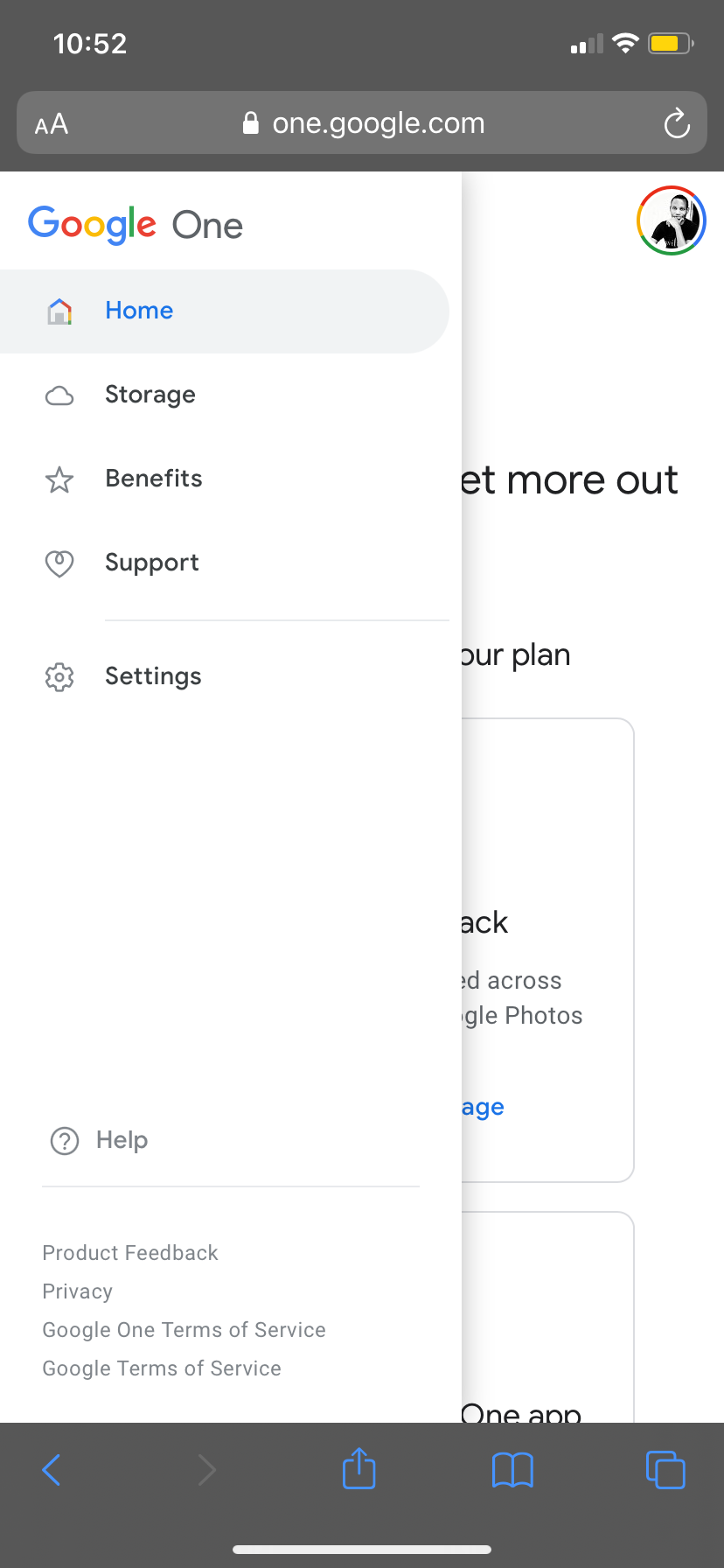The image depicts a smartphone screen in a vertical orientation. At the top, there's a gray status bar showing the time "10:52" on the left, and icons for reception, Wi-Fi, and a yellow battery indicator on the right.

Below the status bar, there's an address bar displaying "1.google.com" with a smaller and bigger capital 'A' icon on the left, a lock icon indicating a secure connection, and a refresh symbol on the right.

Next, the page displays the Google 1 logo, with "Google" in its characteristic multicolored letters and "1" to the right in blue.

Beneath the logo, there is a navigational menu with several tabs. The 'Home' tab is highlighted in blue, while the other tabs include 'Storage' with a cloud icon, 'Benefits' accompanied by a star icon, 'Support' with a heart icon, and 'Settings' marked by a gear icon.

Further down, in gray text, there is a section labeled 'Help' with a question mark inside a circle, followed by links to 'Product Feedback,' 'Privacy,' 'Google 1 Terms of Service,' and 'Google Terms of Service.'

On the right side of the screen, some text is partially obscured by a vertical tab on the left-hand side. At the very bottom of the screen, a gray bar features several blue icons including an arrow, a bookmark, a book, and a multi-tab icon.